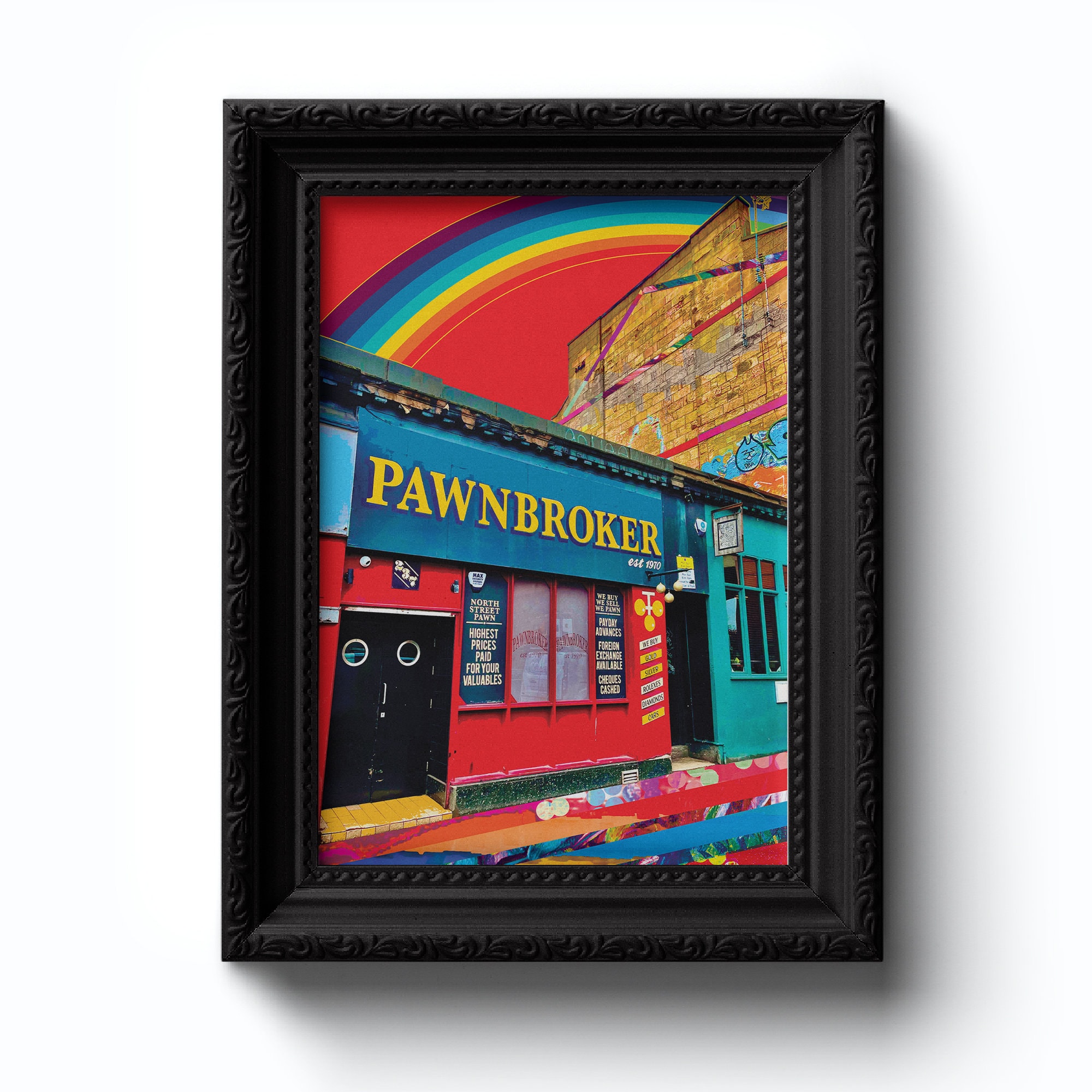The image showcases a framed piece of art with an intricately designed, thick, bold black frame featuring detailed engravings on the outer and inner layers, and a smooth middle layer. The framed artwork is predominantly red and blue, depicting the front facade of a storefront. Central to the image is a red building with a blue banner displaying the word "Pawnbroker" in bright yellow capital letters. The building features two black doors with keyhole windows and four windows beneath the sign, some of which are covered with film or advertisements.

Adjacent to the main building on the right is a turquoise structure, above which a graffiti-adorned brick wall is visible. The sky is vibrantly painted red with an arching rainbow overhead, adding a whimsical touch. The picture is placed against a white background and casts shadows to the right side and the bottom, enhancing its three-dimensional effect. At the bottom right corner of the framed art, colorful bars add an additional splash of vibrancy, completing the overall theme of urban storefronts enlivened by artistic elements.